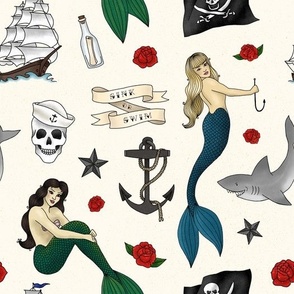The brightly lit piece of artwork features a diverse array of objects intricately positioned against a white background. At the center-right and bottom-left, two mermaids capture attention: the mermaid on the bottom left is crouched in a fetal position, her upper body showcasing flowing brunette hair and Caucasian skin, while her lower half, adorned with green fins and scales, reveals her aquatic nature. The second mermaid, on the center-right, stands with her back to the viewer; she has long blonde hair with bangs, Caucasian skin, and dark blue fins and scales. 

A profusion of other items further enrich the scene. A formidable shark resides on the right, while vibrant red roses, numbering four or five, are scattered throughout. The upper left corner harbors both a seafaring ship with prominent white sails and a bottle containing a message. Adding an element of pirate lore, a black flag with a Jolly Roger and two crossed swords flutters conspicuously. Centrally placed is a charcoal-colored anchor encircled by a ribbon that reads "sink or swim." The visual ensemble is completed with a skull wearing a sailor’s hat and two black stars, lending a whimsical yet nautical theme to the composition.